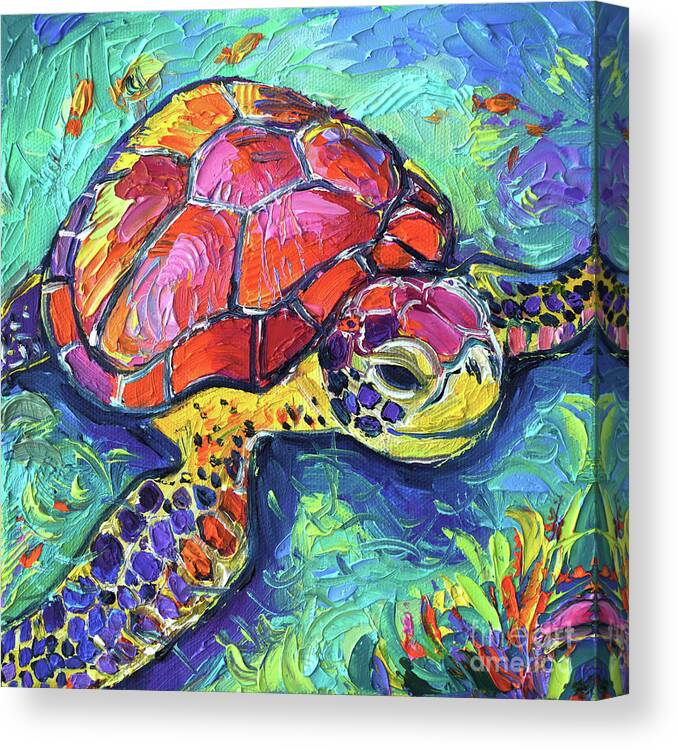This vibrant painting portrays a beautifully detailed turtle, rendered in a pastel or watercolor style with rich texture that mimics oil paint. The turtle takes center stage, showcased in a vivid array of colors: its shell transitions from an orange-reddish hue to a yellowish tint towards the back, and its head's scales match the shell's orange-maroon tones. The turtle's body is mainly yellow, but it features a stunning mix of purple and bluish scales, with darker blue outlines accentuating the intricate details of its face and shell. The background suggests an underwater setting, with greenish-blue swirls implying the movement of water, complemented by hints of vegetation and foliage in the bottom right corner. Beneath the turtle, a cluster of colorful flowers—green, orange, and blue—adds a delightful touch, and the painting's 3D effect is emphasized by the border visible on the left, indicating it is mounted on a box.